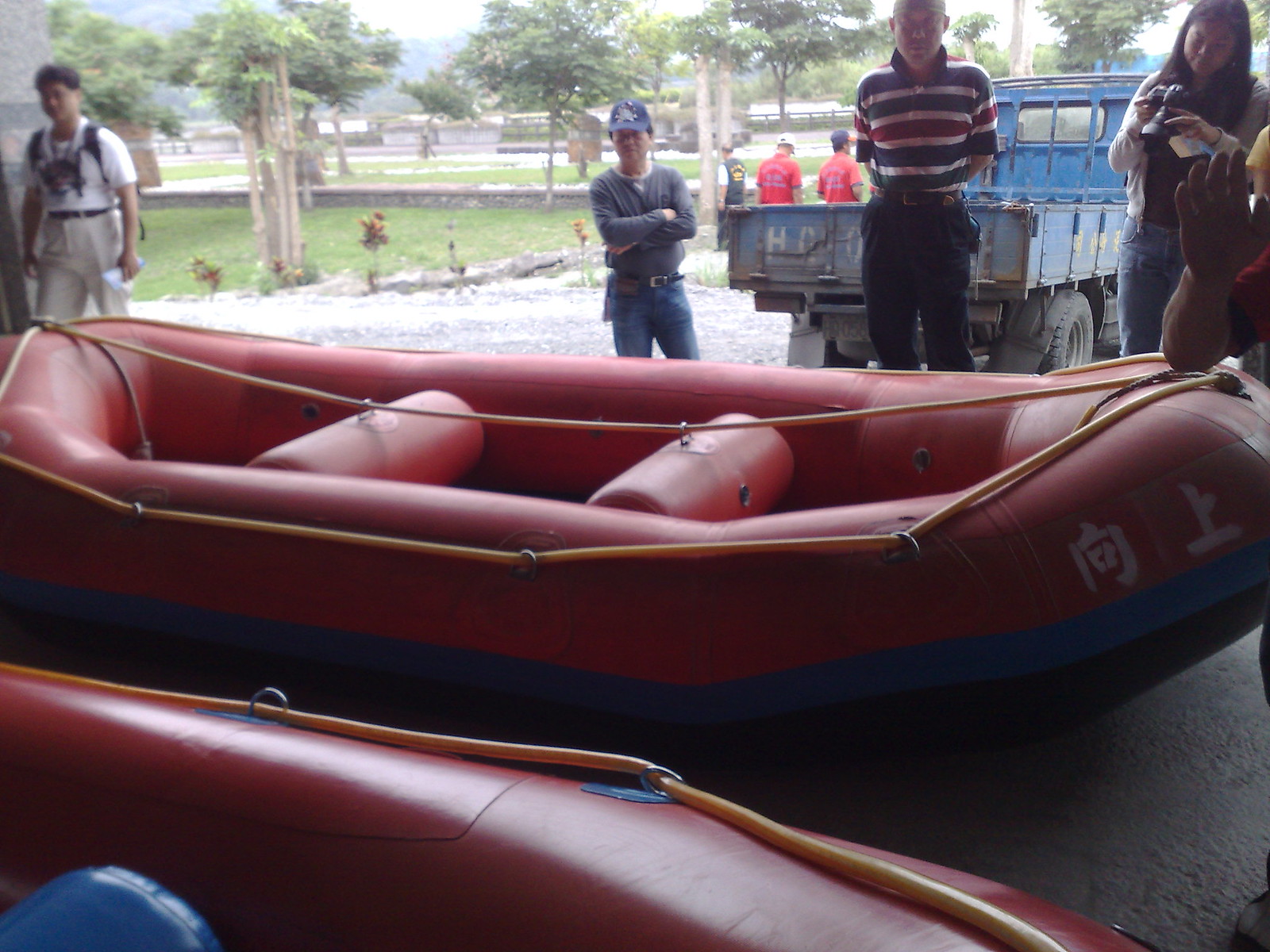This detailed photograph captures a group of people gathered around two large, red inflatable rafts, seemingly preparing for a rafting adventure in a location that appears to be in Mexico, suggested by the people and environment. The rafts are prominently displayed in the foreground, showcasing a curved boat structure with elevated bow and stern, and they contain multiple compartments separated by inflatable benches or structural rods. The rafts are well-equipped with rings across the top sections and a securely fastened rope running along the entire perimeter, indicating durability and readiness for water activities.

In the upper left corner of the image, a man in a white t-shirt stands next to another man with a blue hat and crossed arms, donning a long-sleeved shirt. Central to the group is a man in a distinctive blue, white, and red striped polo shirt with a shaved head, hands behind his back, standing near an old blue flatbed truck. On the right side, a woman is seen focusing on a camera, possibly setting up to take a photo. The scene is set against a backdrop of trees and grass, enhancing the outdoor atmosphere. The juxtaposition of the large, reflective rafts and the people around them creates a sense of anticipation, as if they are gearing up for an exciting time on the water.